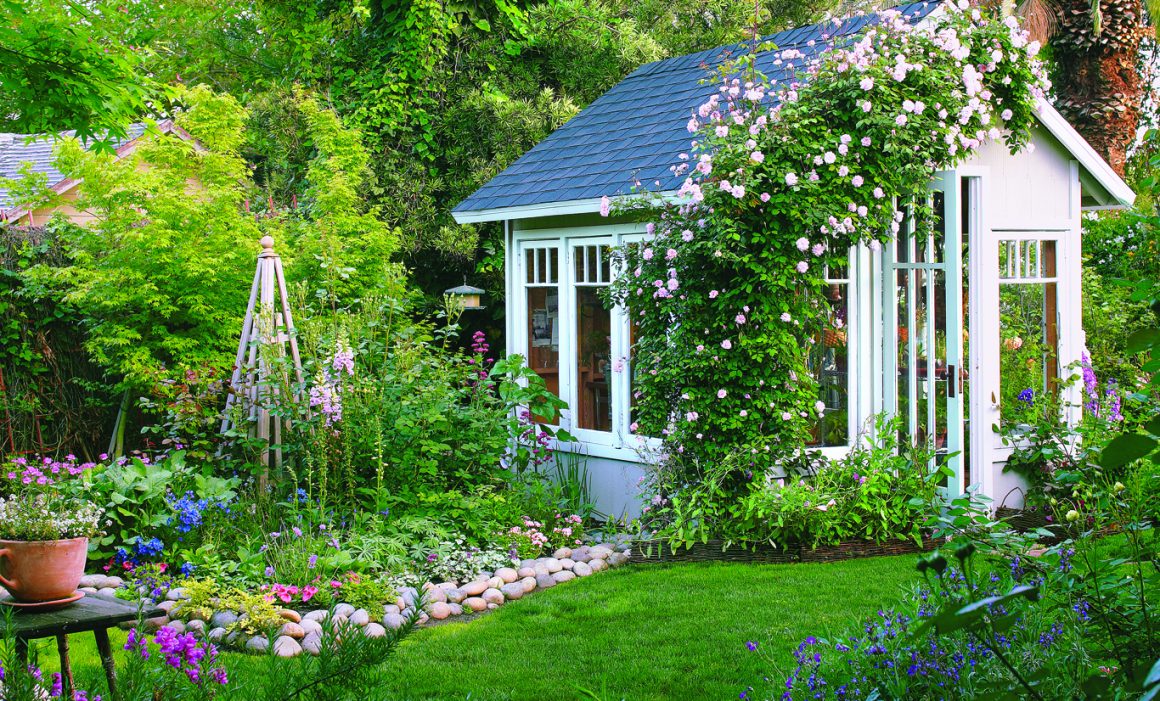The image depicts an outdoor scene showcasing a charming and vibrant little cottage nestled within a lush backyard garden. The cottage, which resembles a tiny house or perhaps an art studio or office, features a gray shingled, pitched roof and numerous windows allowing plenty of light. The exterior of the cottage is adorned with greenery, including large, sprawling vines and various colorful flowers, notably pink ones, which climb around the sides and arch over the windows. A meticulously crafted area, possibly a flower garden, is demarcated by stones and contains diverse plants. On the left side of the image, a table holds a potted plant and a coaster, contributing to the homely and inviting atmosphere. A green lawn stretches out on either side of the cottage, enhancing the vivid, serene environment. In the background, parts of a larger main house and a fence separating this idyllic corner from neighboring properties can be seen. The vibrant and carefully tended flora, combined with the thoughtful architectural details of the quaint cottage, create a picturesque and tranquil garden retreat.